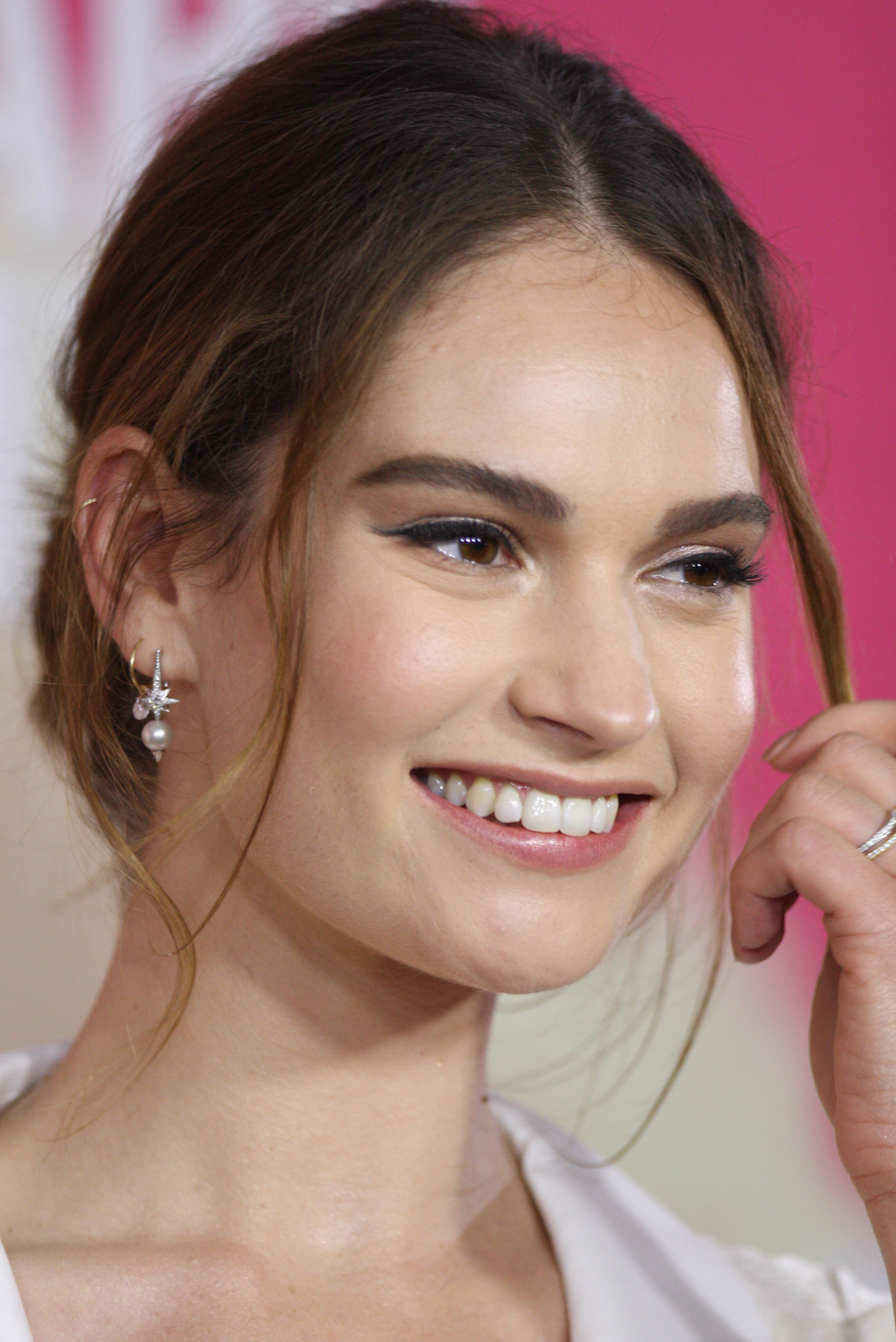This image captures a close-up of a famous actress, resembling Lily James, who appears to be in her twenties. Her brunette hair, accented with chestnut highlights, is pulled back, yet some strands frame her face, and she's holding one between her fingers. Notably, she has two thin diamond rings on her left hand's ring finger, suggesting a wedding band or engagement ring. Her right ear showcases an array of earrings: a dangling earring with a star and pearl, a second hoop earring, and another hoop at the top. She smiles warmly, showing her upper teeth, and looks to the right side, away from the camera. She has brown eyes and her attire includes a white top, possibly a stylish shirt or jacket, visible only at the neckline. The blurred background is pink and white, hinting at a promotional event setting.